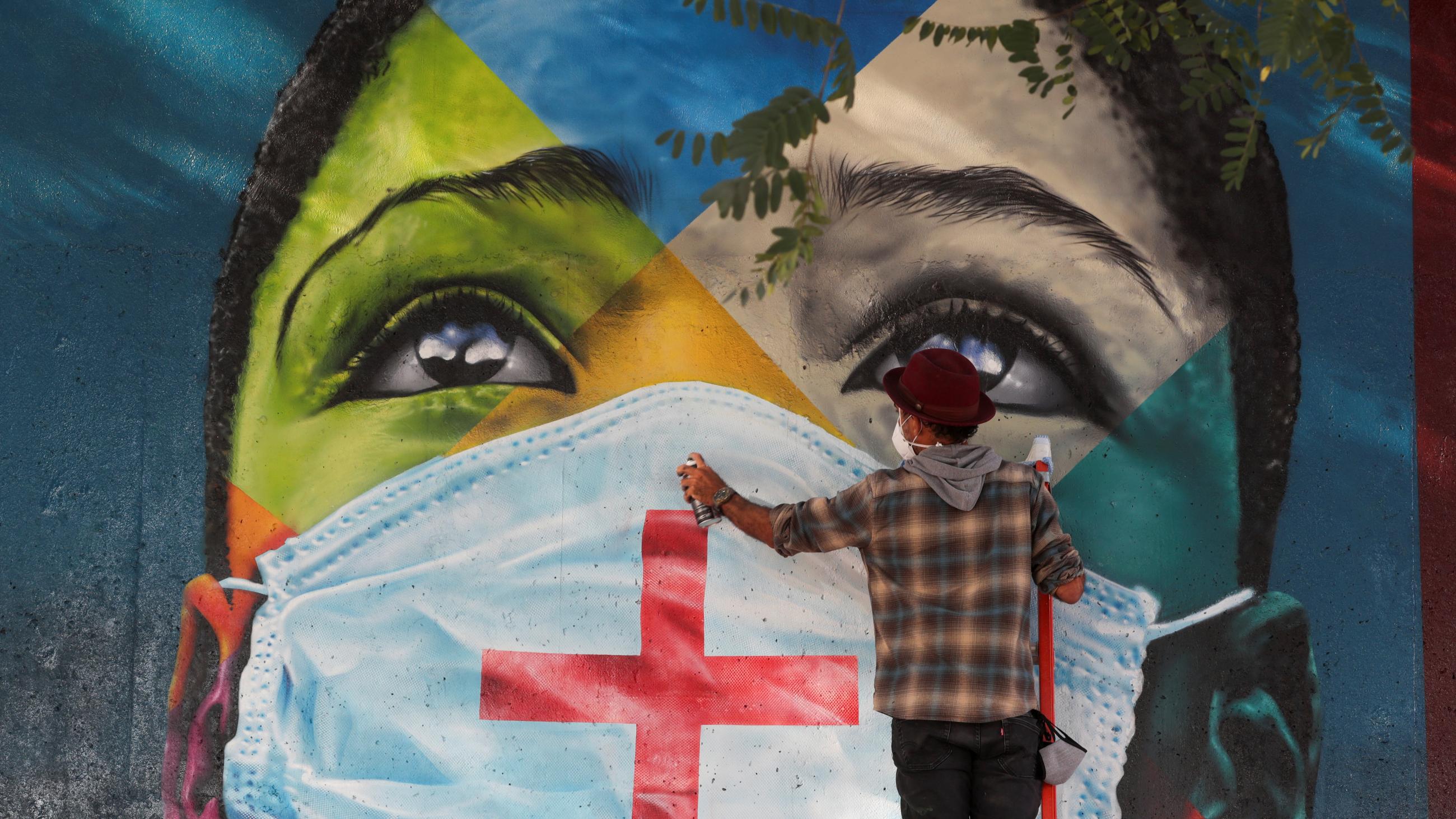The image captures an artist in the process of creating a detailed mural on a wall. The mural portrays a person's head, segmented into four distinct colored quadrants: the top is blue, the left is green, the right is grayish white, and the bottom is yellow. The left and right quadrants focus on the eyes, while the bottom quadrant showcases a nose covered by a white mask with a red cross, indicative of a healthcare theme. The background surrounding the head features varying shades of blue, and on the top left, green leaves and brown stems frame the face. A bold, vertical red line delineates the right side of the mural. 

In the mural, the top of the forehead contains a blue triangle, the right side of the face has a green square, and the left features a gray square. The nose, depicted in the yellow bottom quadrant, has an orange triangle above it. The left side (viewer's right) of the head shows additional blue and orange accents.

The artist, seen from behind, is holding a spray can in their left hand and appears to be positioned on a ladder, implied by their elevated height. The artist is wearing a blue, yellow, and black plaid shirt with sleeves rolled up to the elbows, a black hat, black pants, and a mask for safety. They have a gray hoodie beneath the shirt and a gray and black mask hanging from a belt loop, accentuating their commitment to safety. A gray wristwatch and a burgundy fedora complete the detailed colorful attire of the spray-painting artist, blending them seamlessly yet distinctively into their vibrant creation.